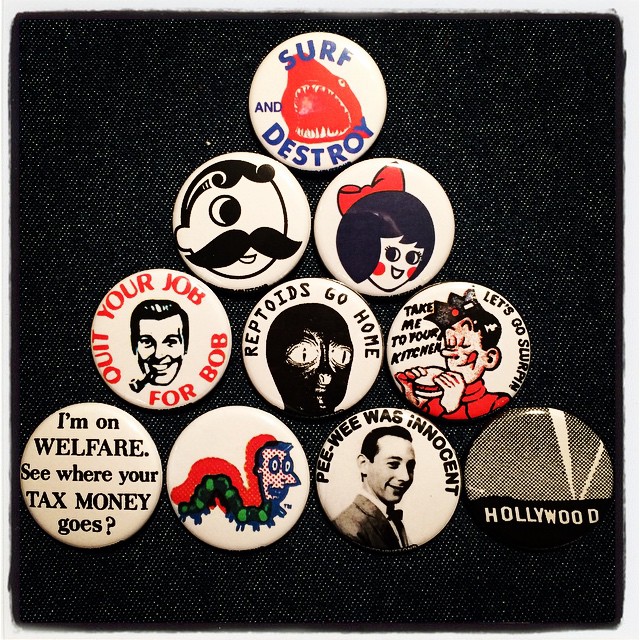This image features a set of 10 round badges meticulously arranged in the shape of a pyramid against a black surface. At the very top, a white badge prominently displays the slogan "Surf and Destroy" along with a vivid red shark head graphic. Below it, aligned in the second row, the left badge portrays a cartoon man with one googly eye, a black mustache, curly black hair, and a wide smile, while the right badge features a cartoon girl with a red bow in her black hair.

The third row from the top includes three distinguishable badges. On the left, there's a white badge with a black-and-white sketch of a man smoking a pipe, accompanied by the red text, "Quit Your Job for Bob." At the center, another badge showcases an alien face with black skin and the command, "Reptoids Go Home," displayed in black font. The right badge in this row illustrates a character eating a sandwich, with the unusual slogan "Take Me to Your Kitchen, Let's Go Slurping," while the character dons a red turtleneck.

The fourth row expands to four badges. From left to right, the first badge declares, "I’m on Welfare, See Where Your Tax Money Goes." Next, there's a badge featuring a caterpillar with a human-like face. Following this, another badge reads, "Peewee Was Innocent," and the final badge of the row simply states, "Hollywood."

This artistic assortment of badges blends text and whimsical graphics, capturing a diverse array of messages and characters.